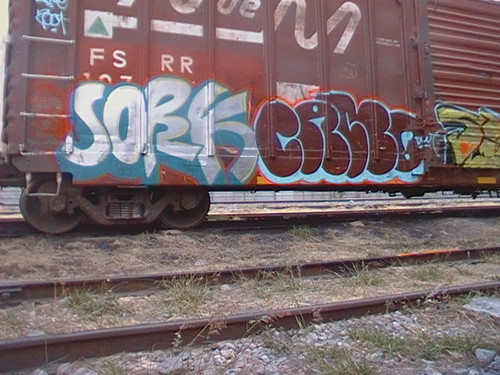This image captures the lower portion of a dark maroon-red boxcar train parked on brown train tracks, surrounded by pebbles, rocks, hay, and patches of yellow and green grass. The wheels of the train are visible on the left side. Prominently displayed on the side of the train car is graffiti in vibrant colors, including white, teal, light blue, and yellow. Among the various pieces, one reads "S.O.B.K.," painted in white and blue, and another section includes the letters "C.R.C.C.O!" in silver, blue, dark purple, light blue, and yellow, suggesting a signature style common in metropolitan areas. The graffiti is positioned within arm's reach, indicating it was likely created by an artist on the ground. There's also smudged text on the train car that says "F.S.R.R.," accompanied by a partially framed-out logo.